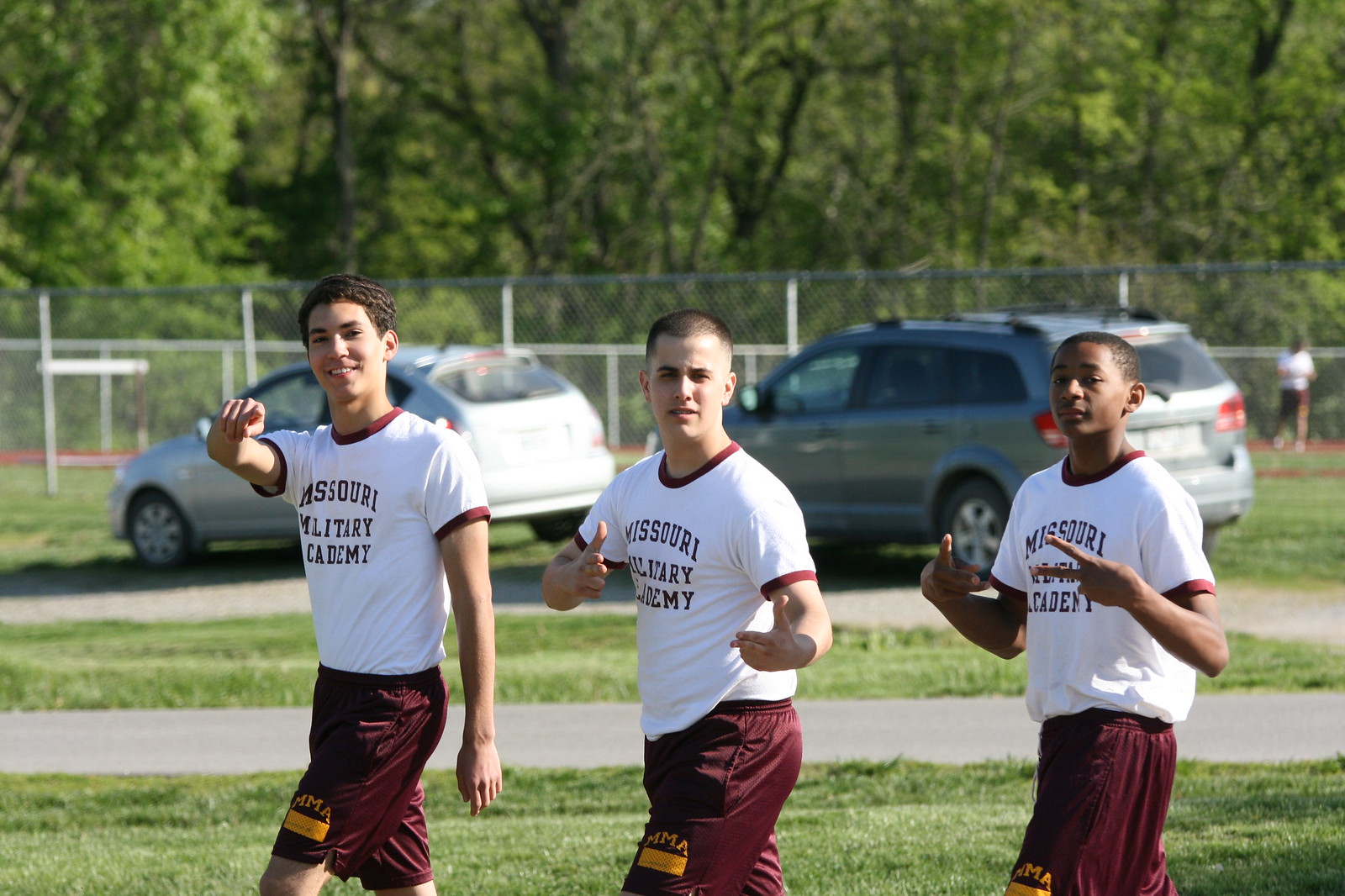The photograph captures three young men posing outdoors on a bright, sunny day. They are dressed in matching uniforms consisting of cranberry-red shorts with the gold letters "MMA" and a yellow rectangle on the front. Their white short-sleeved T-shirts feature dark purple lettering that reads "Missouri Military Academy" and have cranberry hems around the sleeves and collar. Each young man is engaging with the camera through distinct hand gestures: the leftmost is pointing with his index finger, the middle one is making finger guns, and the rightmost is flashing a double peace sign. The background reveals a tree-lined area with greenery and two vehicles, a light blue SUV, and a light gray hatchback, parked along a gravel path near a chain-link fence. The setting appears to be a slightly wooded area with visible paved roads and a walking path. The prominent colors in the image are green, white, purple, and light blue.